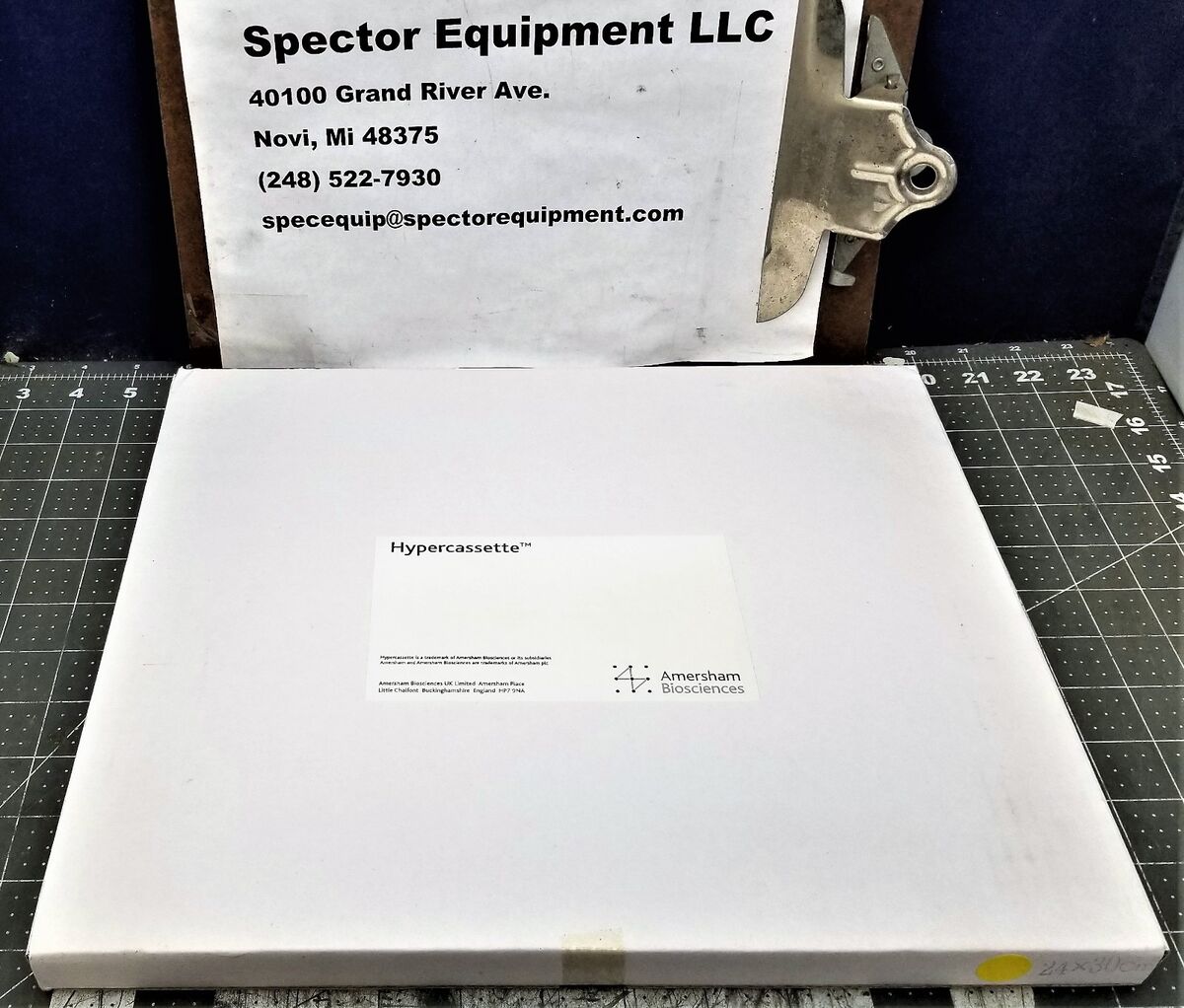The image showcases a meticulously arranged scene featuring a measuring mat with numbers and grids, positioned centrally against a dark blue wall. Dominating the center of the mat is a package identified as a "HyperCassette™," prominently labeled with the logo of Amerisham Biosciences. The white package, approximately 15 cm wide, remains unopened. Positioned directly behind the package is a clipboard leaning against the wall, holding a paper with the header "Spectre Equipment, LLC," listing contact details including the address 40100 Grand River Ave, Novi, MI 48375, the phone number 248-522-7930, and the email SPECEQUIP@SPECTOREQUIPMENT.COM. The overall composition highlights the alignment of the package and the clipboard, creating a balanced and structured visual presentation.